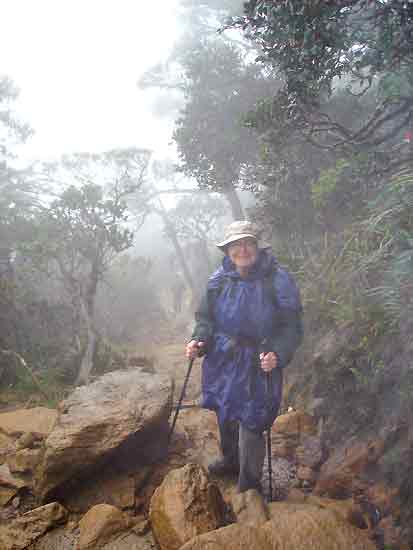This photograph captures an older woman, possibly in her 60s or 70s, during a hike through rocky terrain. She is equipped with two hiking poles and dressed in a blue or purple rain jacket, indicative of the misty or rainy weather. Her tan, wide-brimmed hat shields her face from the elements. The woman stands confidently amidst large, muddy brown rocks, the largest of which is about waist-high and slightly wider than her. The rocky path she's on is surrounded by an assortment of trees and plants, with various branches and leaves visible, some even appearing green or purple. The background reveals more trees and a sense of depth created by the misty or rainy atmosphere, which softens the distant view. To the right, there are additional plants and leaves hanging off, contributing to the lush, almost jungle-like feel of the scene. Gray clouds loom overhead, enhancing the dreary ambiance. There is also a hint of another person in the distance, further along the trail.